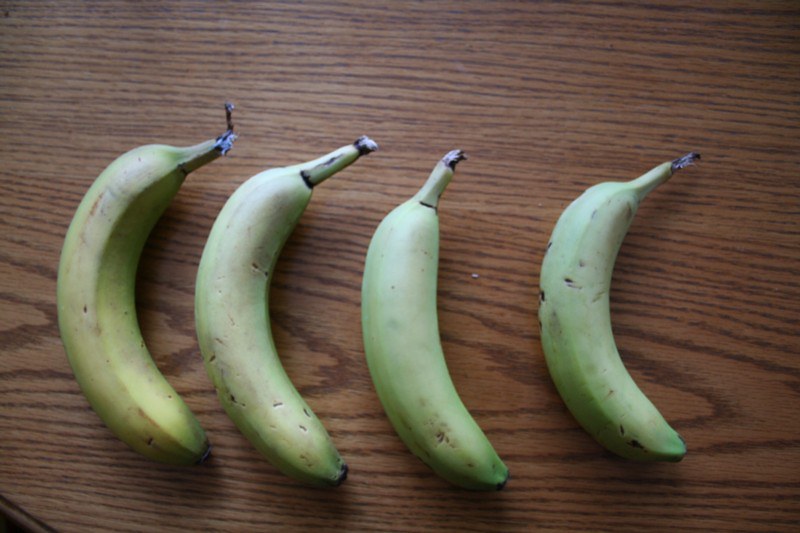Four unripe bananas lie gracefully on a finely-grained wooden table. The table's surface is predominantly adorned with narrow, uniform lines, except for a central section beneath the bananas where the grain widens, hinting at the inner rings of a tree. This wider pattern offers a contrast to the otherwise delicate wooden texture, illuminating the tree's growth rings in a broader, more pronounced manner. The green bananas are sprinkled with minor black spots and show signs of slight bruising, indicating they have been handled. The banana on the far left is beginning to show hints of yellow and has a small break at the stem, unlike the other three, whose stems remain largely intact. Despite their current unripeness, these bananas hint at a brief window of ripeness before over-ripening. In the corner of the image, a tiny, indistinguishable object peeks in, adding an element of intrigue to this otherwise serene still life.